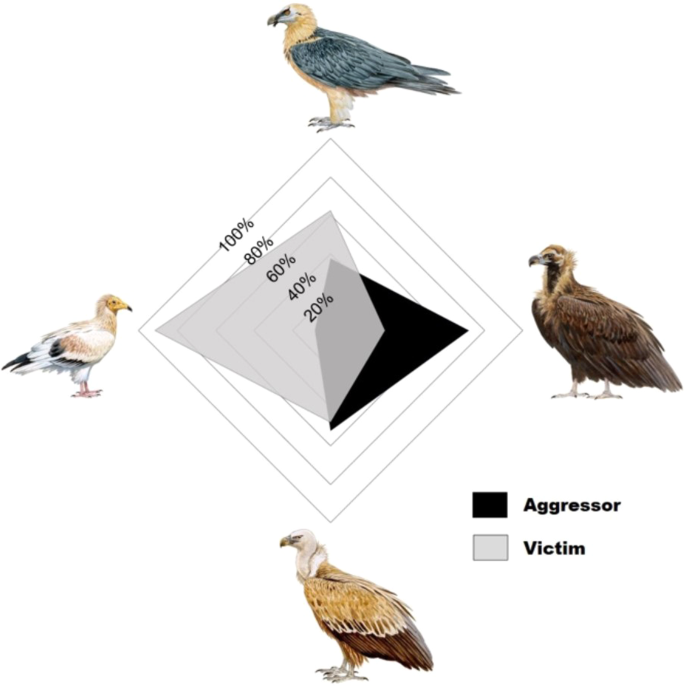The image is a detailed diagram featuring four distinct birds positioned around a central diamond-shaped graphic. Each bird occupies a top, right, bottom, or left corner. The top bird has a white face, brown body, and gray wings and tail, associated more with victim characteristics. To the right is another bird, predominantly brown, with features aligning more with aggressor traits. The bottom bird showcases a white head with a mix of light and dark brown wings. The left bird exhibits a mix of white, black, and brown plumage with a yellow beak tipped with black, depicted strongly as a victim.

At the center of the diagram is a graphic composed of concentric diamonds or squares with descending percentages labeled 100%, 80%, 60%, 40%, and 20% towards the inside. The interior shapes are shaded in gray tones indicating different roles; light gray for victims and dark gray for aggressors. A key to the right of the diagram identifies these roles using gray and black squares with accompanying text. The diagram effectively uses color coding and positioning to illustrate the distribution of aggressor and victim traits among the pictured birds.